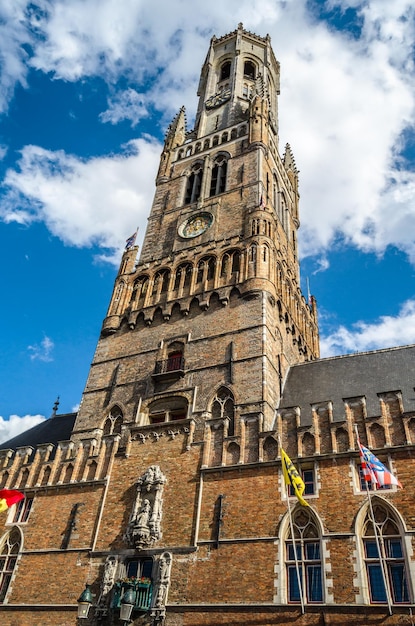This outdoor photograph captures a majestic brownstone or brick building with a towering, multi-storied structure. Taken from a kneeling perspective, the building appears to loom grandly against a blue sky dotted with white, wispy clouds. The building showcases three arches on the first floor and several arched windows, possibly stained glass, framed by lighter colored stone. Dominating the image, a colossal cylindrical tower, flanked by turrets and transitioning into an octagonal top, stretches skyward. Midway up the tower, a clock face is visible. Below the arches, three flags flutter in the foreground: one red, white, and blue, another yellow and black, and a third, red and yellow. A doorway, topped by a statue, adds to the regal architectural elements, while the gabled roof contributes to the building’s imposing and historical presence.